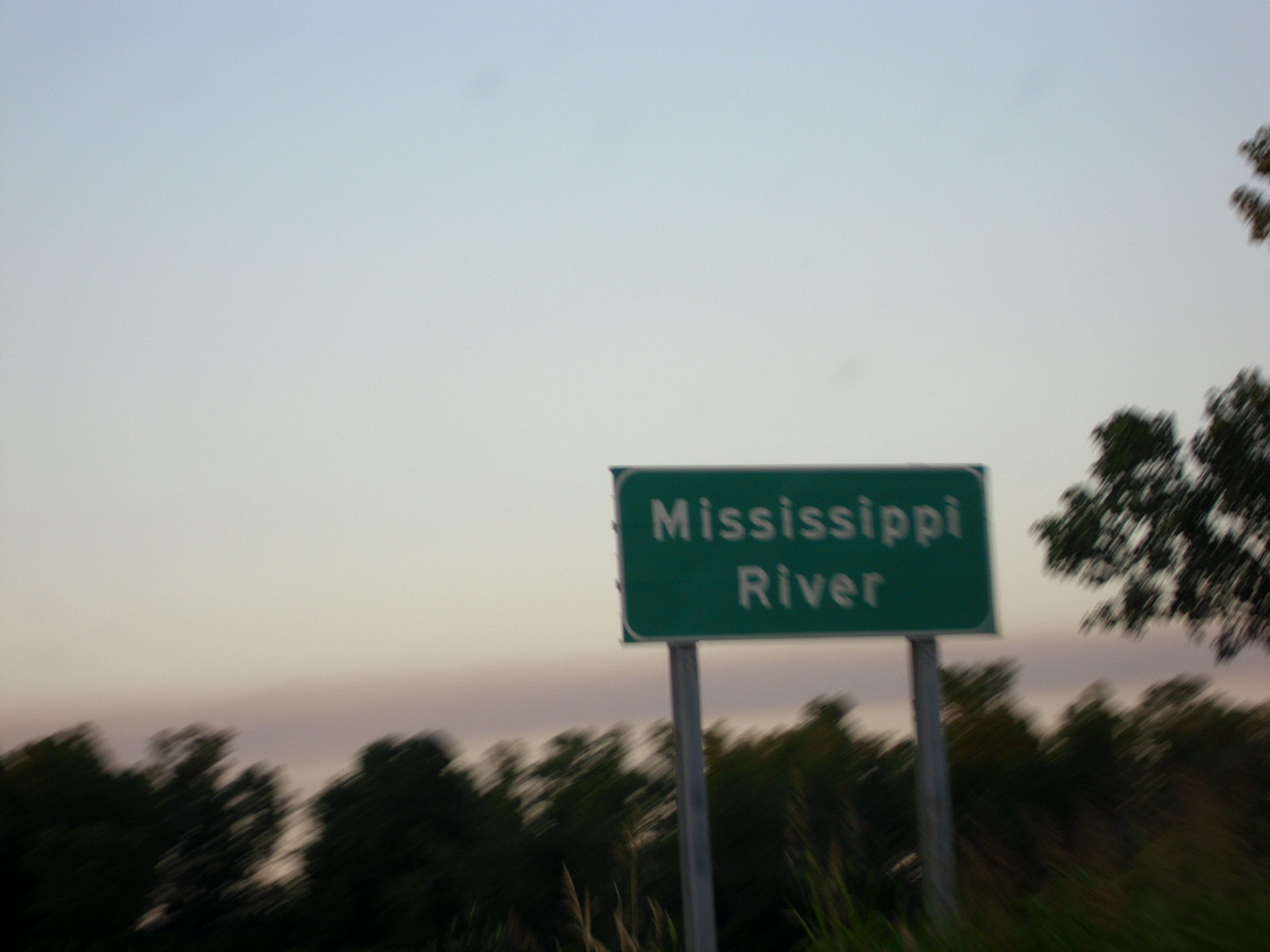The photograph captures a green sign mounted on two steel posts by the side of a highway, with the white text "Mississippi River" centered on the sign. The image, though slightly grainy and artistic, shows an overgrown foreground of lighter green grass with hints of brown. In the background, thick, leafy green trees are visible, albeit with some blurring motion. The sky transitions from a partially blue hue at the top, with faint hints of pale pink and purple blending into a creamy yellow and pale grayish-purple about three quarters down the photo. Off to the right side, several branches with green leaves protrude into the frame, adding to the overall lush, natural ambiance of the scene.